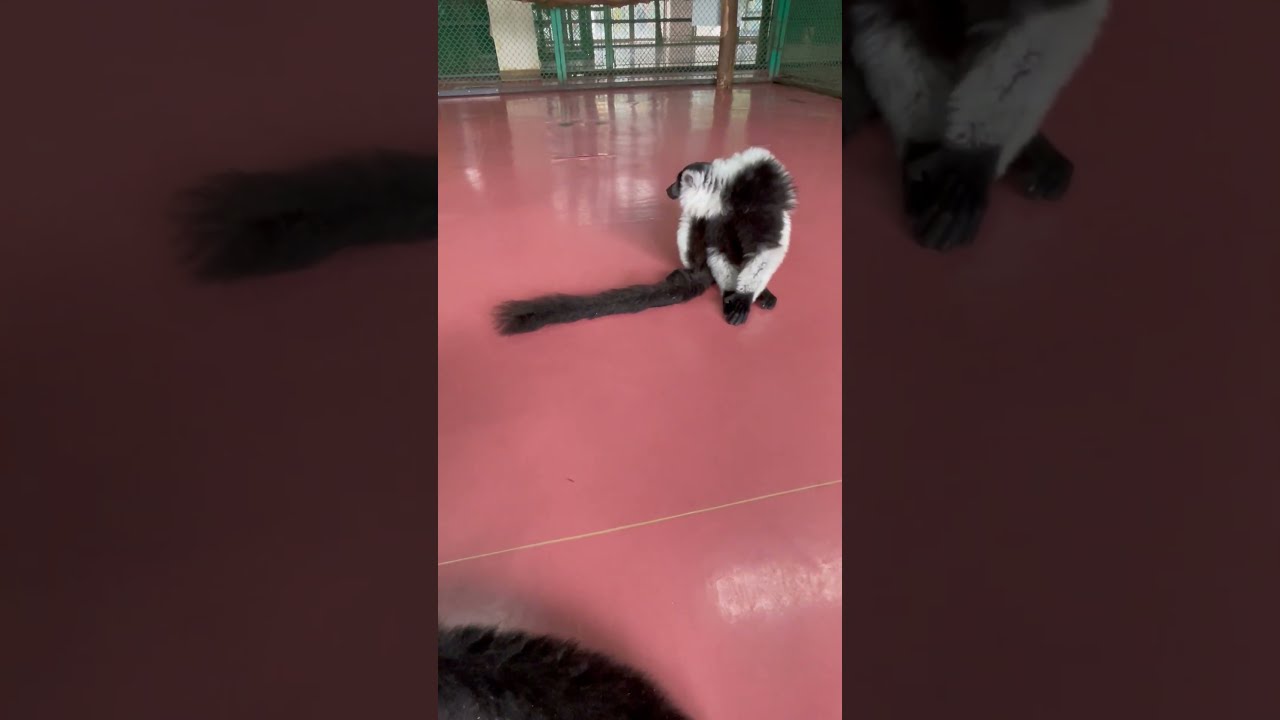The image shows a black and white mammal, potentially a lemur or a skunk, with a long, bushy black tail and a pointed snout. The animal is positioned on a pinkish-reddish, polished concrete floor that reflects light, suggesting a hard surface. It appears to be inside a larger caged area, defined by green metal fencing and a silver gate visible in the background. There are no other discernible animals or people in the scene, though some darker brown elements frame the sides of the image. The setting looks like an indoor enclosure, possibly part of a zoo exhibit.